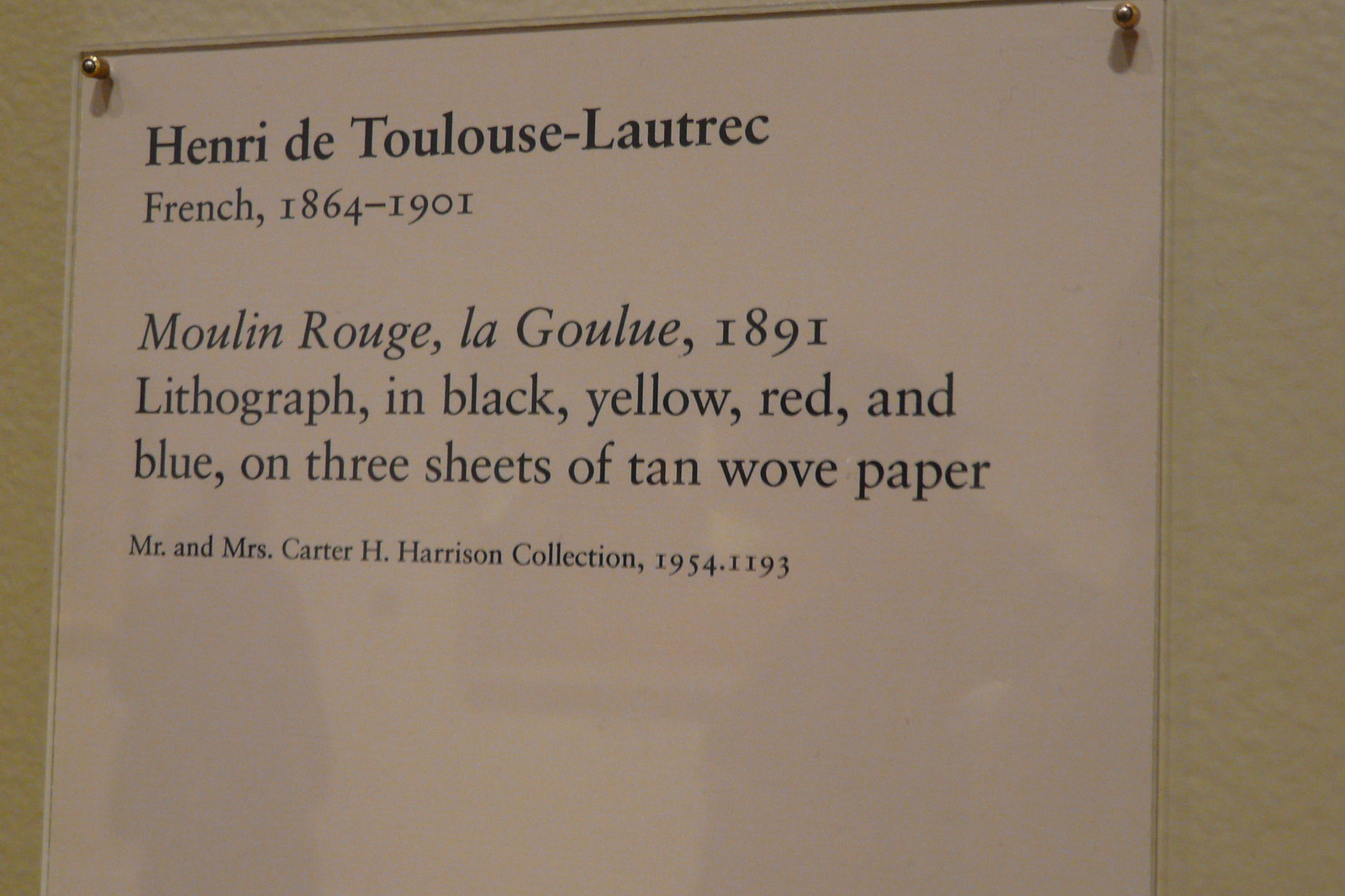This indoor photograph, shot in landscape mode, showcases a museum or art gallery description card, affixed to a white wall. The description card, a white elongated rectangle, is encased in clear plexiglass, revealing slight reflections of people. At the card's top corners, small pins or screws secure it to the wall. The card's bold black text begins with "Henri de Toulouse-Lautrec," followed by "French, 1864-1901." Below are the details of the artwork: "Moulin Rouge, La Goulue, 1891," described as a "lithograph in black, yellow, red, and blue on three sheets of tan wove paper." At the bottom, in smaller black text, it credits the "Mr. and Mrs. Carter H. Harrison Collection, 1954-1193." The photograph captures only the placard, without the accompanying artwork.